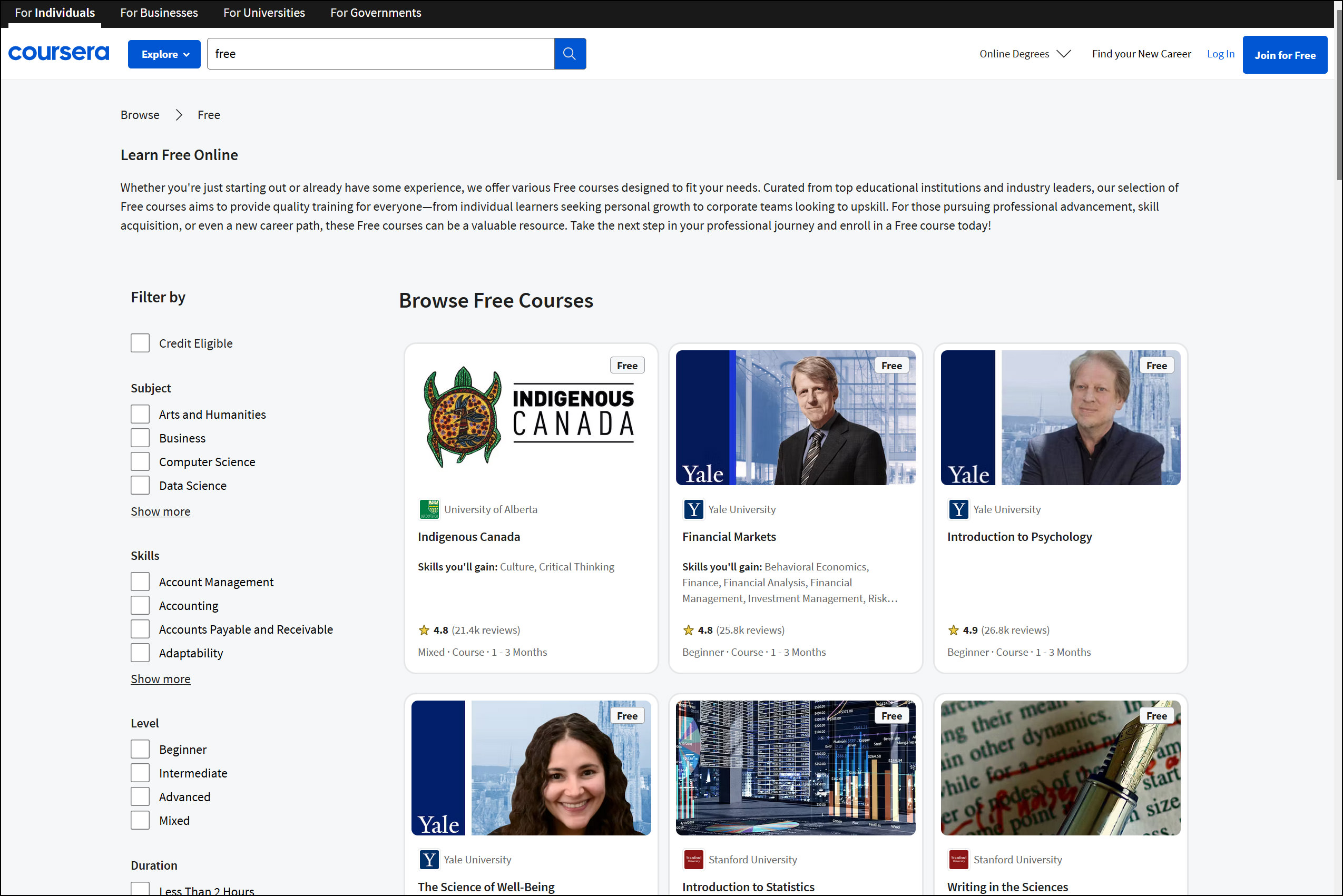This is a detailed screenshot of the Coursera website interface. The image features a rectangular layout with a light gray background throughout. In the upper left corner, "Coursera" is written in blue text. At the top of the screenshot, a black menu bar with white text displays several clickable tabs labeled "For Individuals," "For Businesses," "For Universities," and "For Governments." 

Below the menu bar, there is a white search bar outlined in medium gray, containing a search query that reads "free." On the left side of the search bar, there is a drop-down menu button labeled "Explore" in white text, while the right side features a small square icon with a blue background and a white magnifying glass in the center.

Under the search bar, informative text indicates the availability of free online learning. To the right, there is a section titled "Browse Free Courses," displayed in black text. Below this, previews of various courses are visible. The first course on the list is titled "Indigenous Canada," marked as free. Each course preview in the upper right corner has a small white button with a gray outline labeled "free."

On the left side of the screenshot, there is a filter section with checkboxes to refine search criteria, making it easier for users to select their desired courses.